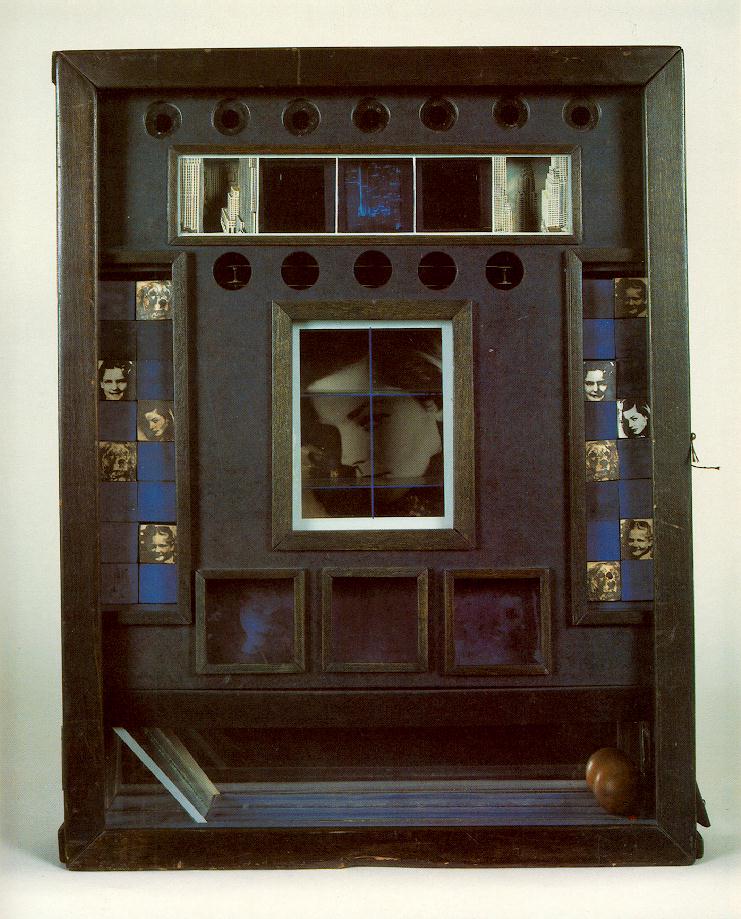The artwork features a complex and ornate wooden frame, primarily brown with hints of a faded brownish-green. The frame encompasses a central black-and-white photograph of a woman's side profile, surrounded by various smaller photographs. These smaller images, also in black and white, depict buildings, women's faces, and a dog, likely of sentimental value. The overall shape of the artwork is more squared than it is tall, and it includes several noteworthy elements: squares within squares and a series of circles at the top. Specifically, five circles are aligned horizontally in the upper middle, with seven more circles at the very top of the piece. Flanking the central photograph are sections with vertical blue strips that contain additional smaller photo slots. The left and right sides each feature a checkerboard-like pattern with diagonal arrangements of images and empty slots. At the bottom, there is a peculiar section with a doorknob and a ramp or slide-like feature, adding an element of mystery to the piece. The entire artwork rests against a white background, enhancing its intricate details and design.